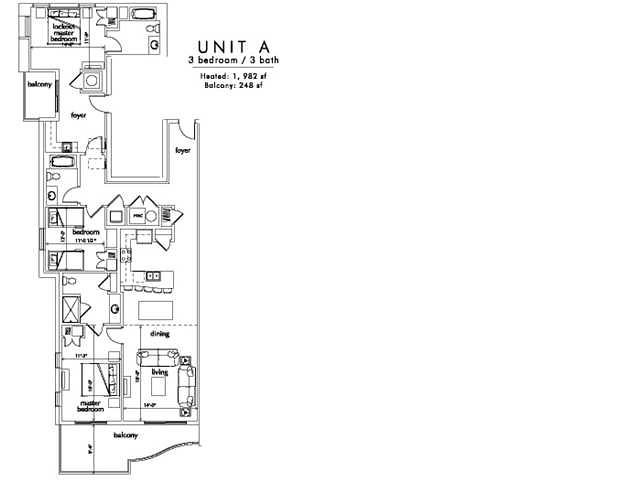This is a blueprint of "Unit A," a single-floor residence. The layout features three bedrooms and three bathrooms. Due to the small size of the print, some details are difficult to decipher. However, the blueprint appears to indicate heated spaces and room dimensions. The residence includes a cozy balcony accessible from both the living room and one of the bedrooms, which provides a seamless indoor-outdoor living experience.

Upon entering Unit A, there is a foyer that leads into the main living areas. The living room and dining space are adjacent to the balcony, creating a communal area that flows into the kitchen. The kitchen is equipped with a bar stool countertop, providing an informal dining option or a space for social gatherings.

The layout also comprises three bedrooms, each conveniently located near a bathroom. The first bedroom faces the balcony along with the living area, enhancing the room's natural light and accessibility. The second bedroom is situated near the dining space, while the third bedroom is located towards the back, farthest from the balcony, ensuring privacy. Each of the bathrooms is strategically placed to serve the occupants effectively. Overall, Unit A is designed to maximize both communal and private spaces within its compact footprint.